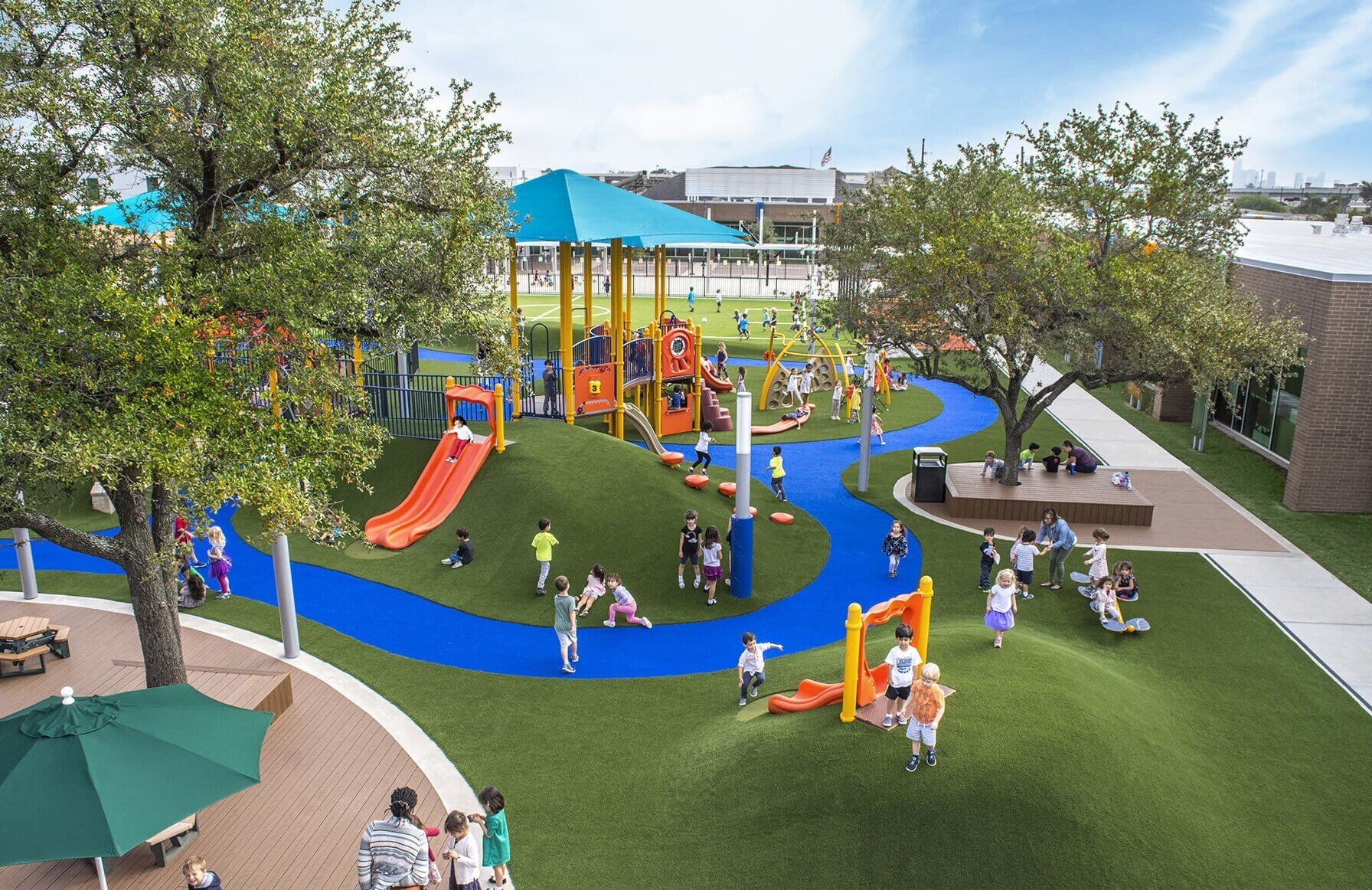This image is an aerial photograph of an idyllic and highly detailed children's playground, potentially located on school grounds. The central focus of the playground features a large, paired plastic slide, surrounded by various other play structures and a vibrant blue pathway that wends its way through the play areas, resembling a river. The ground, covered in what looks like artificial green grass, contrasts with the vivid blue trail. Dotted throughout the playground are numerous children and a few adults engaged in play and activities.

Towards the bottom left of the image, a brick-paved patio area provides a place to rest, complete with green umbrellas and picnic tables. In proximity, a live oak-looking tree stands tall, adding natural beauty to the scene. Additionally, there are seating areas ingeniously incorporating brick structures with planted trees, surrounded by other similar rest sections. 

Buildings frame the playground on the sides and rear, creating an enclosed, safe environment. The layout also includes a blue sky with fluffy white clouds scattered above, enhancing the serene yet lively atmosphere of this recreational haven.